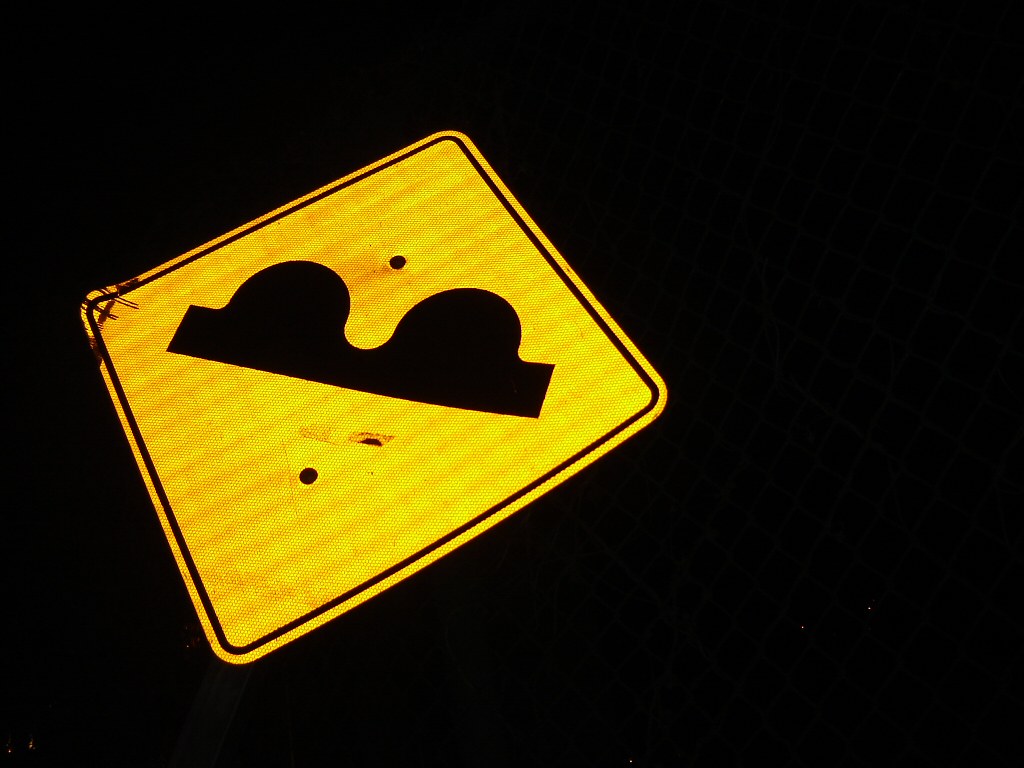The image depicts a yellow highway sign, shaped like a diamond when oriented at certain angles, but it can also resemble a square. The sign has a dark brown border and features a black symbol in the center. The symbol, which could be interpreted in several ways, resembles two breasts or humps when viewed upside down or from a different perspective, it might look like the letter "B". Additionally, there are two dark spots on the sign, possibly resembling holes. One of the corners of the sign appears to have some paint or another substance on it.